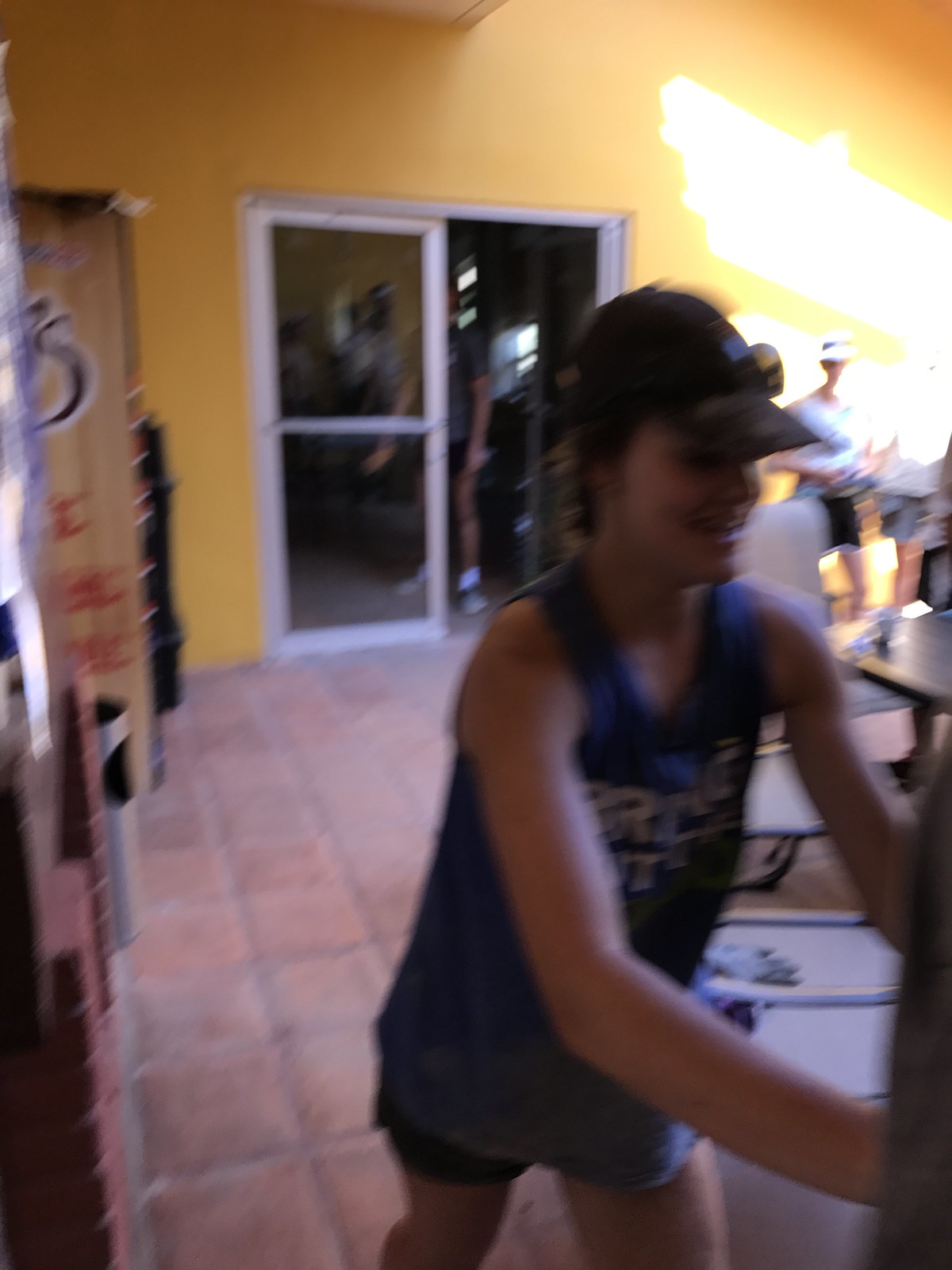This photograph captures a scene that, although out-of-focus, conveys a casual moment. At the center stands a girl, clad in a long T-shirt and short shorts. She accessorizes with a black hat, onto which she has perched a pair of sunglasses. She appears to be interacting with a soda machine on the right side of the image, though the exact action is indistinct. The floor beneath her feet is covered in terracotta square tiles, adding a rustic charm to the setting. Behind her, a yellow wall is bathed in sunlight streaming from windows above, highlighting the warm tones of the space. To the left, there is a stack of bricks, while on the right, a large glass and aluminum door, comprising two doors, stands prominently. The photo evokes a sense of everyday simplicity amidst a vividly illuminated setting.